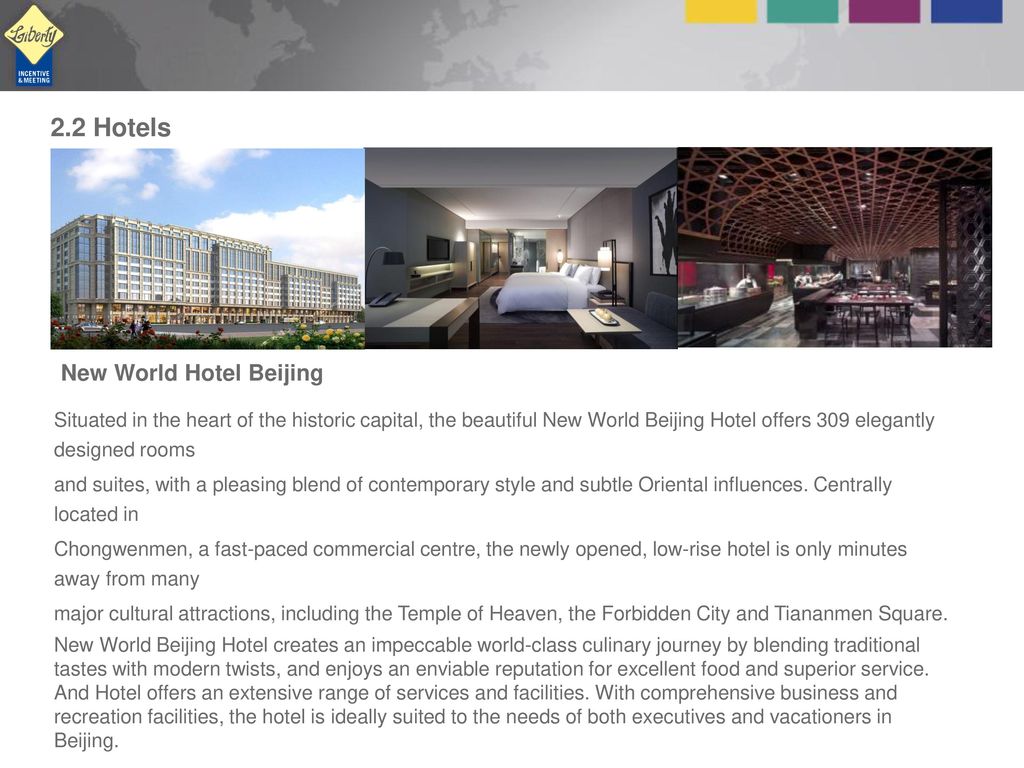The website for a hotel in Beijing targets world travelers, offering a modern and elegant choice for their next stay. At the top of the site, a sleek gray bar is adorned with a faintly visible world map as a background feature. This design element adds a global touch, symbolizing the hotel's international clientele. Placed prominently within this gray bar are four colored boxes—yellow, green, purple, and blue—which serve as part of the hotel's unique branding, despite not having direct functional significance on the site. 

The hotel's logo, a subtly designed pale-colored diamond atop a blue box, is also featured in this section. Just beneath the gray bar, the slogan "2.2 Hotels" is displayed, although its precise meaning remains unclear.

Following the slogan, the website showcases three inviting images of the hotel. The exterior view reveals a contemporary low-rise building, exuding both modernity and sophistication. The interior images highlight spacious and stylish rooms, along with a beautifully designed restaurant, promising a luxurious and comfortable stay for guests.